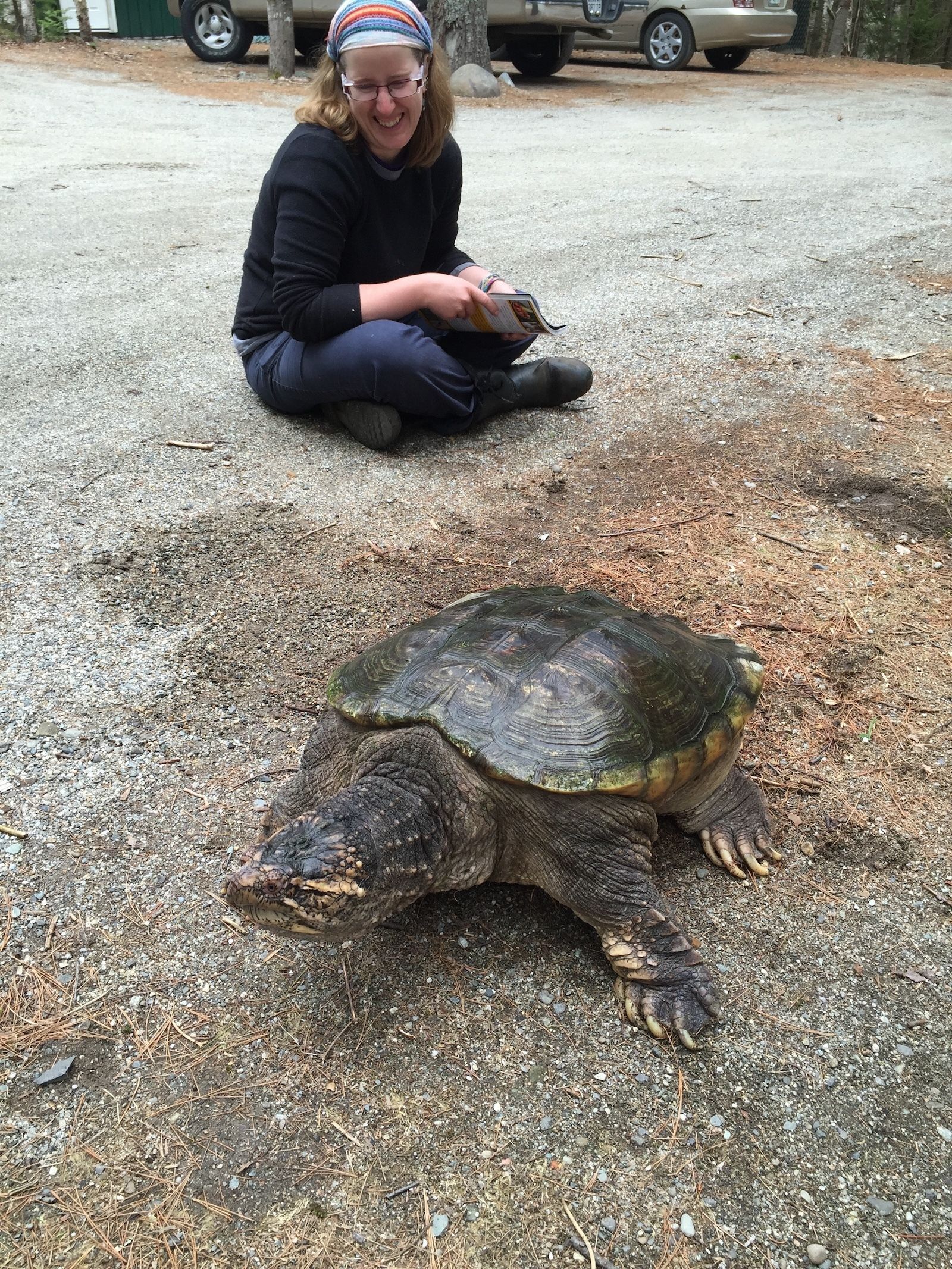In this outdoor photograph taken in a natural setting, the main focus is on a large tortoise with a green shell and brown body and legs, positioned at a 45-degree angle towards the camera. The tortoise is standing on the edge of an unpaved, rocky road scattered with pine needles and leaf litter. Nearby, a woman with fair skin, blonde hair, and glasses is sitting cross-legged on the dirt ground, wearing a white, red, and blue headband, a black long-sleeved shirt, and navy pants. She is holding a magazine or booklet, looking down at the tortoise and laughing. The scene also includes a glimpse of two parked cars in the background. Her body language and expression suggest she is amused by the tortoise, which appears to be slowly walking away from her.